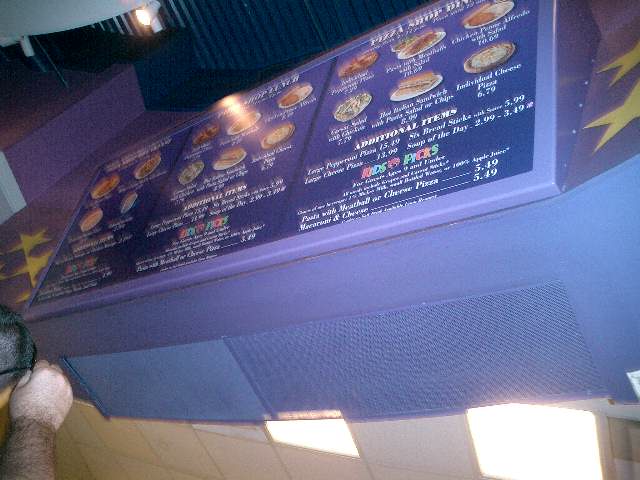The photograph depicts the interior of a pizza shop. Central to the image is a large menu displayed above the kitchen area. The menu is set against a medium blue cabinet, with the writing appearing on a darker blue background. Surrounding the sign are some yellow stars, two or three on each side, enhancing the decor.

Above the menu, there is a metal structure with a rippling effect, also in blue. In the lower left corner of the photo, a white hand is visible, reaching up to grab something. The arm, starting from the wrist, is in the shadows but appears to be hairy and dark.

The text on the menu is mostly unreadable, though the words "Pizza Shop" and "Additional Items" are discernible. The top row of the menu features different circular images, possibly representing plates with various offerings. Below this section, the items are listed under "Additional Items," though their exact descriptions are not clear. The next section, titled "Kids' Picks," shows items priced at $5.49. The middle section of the menu seems to follow a similar layout.